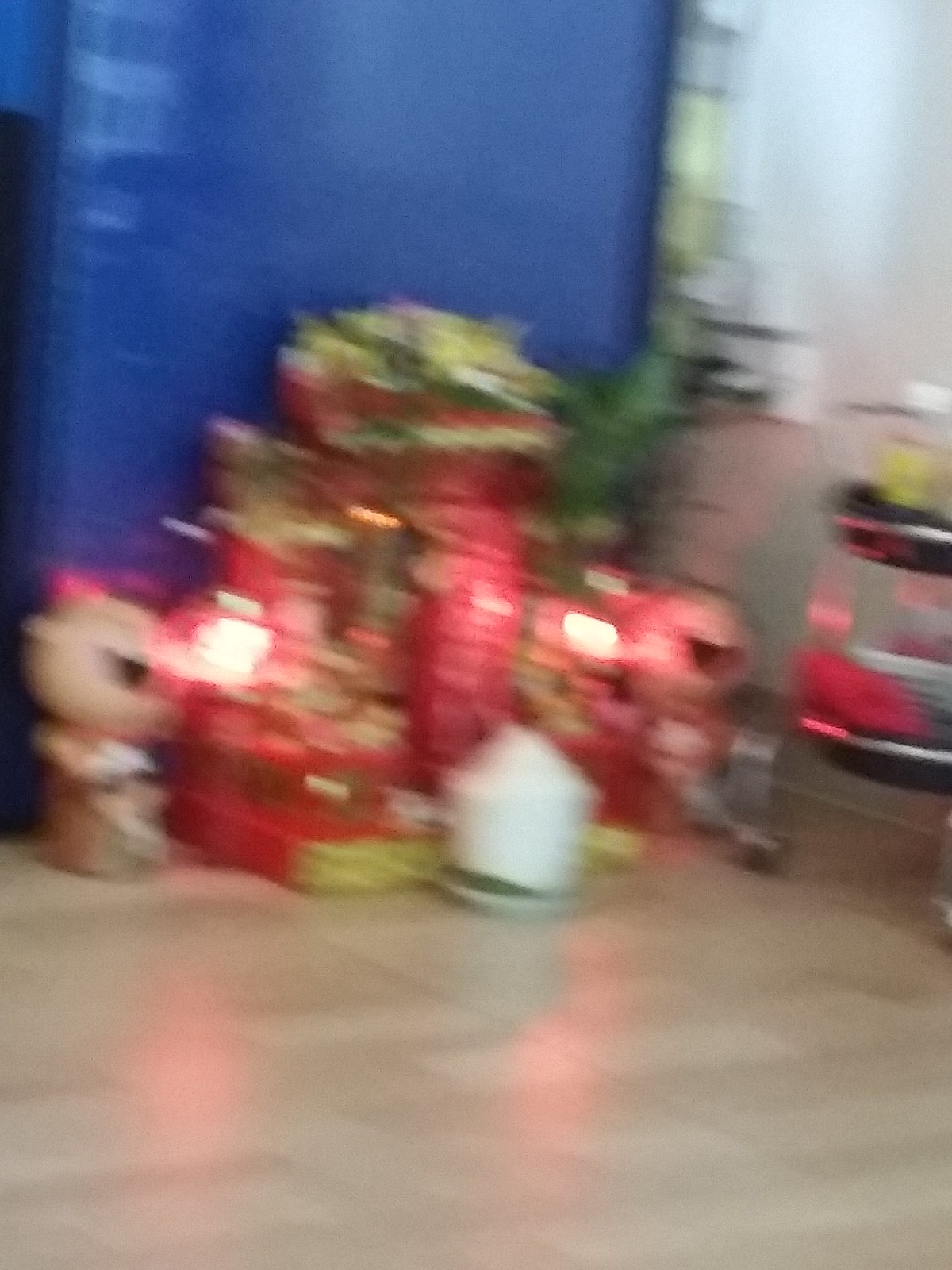The very blurry image reveals a central arrangement of red and white objects, possibly parcels, adorned with some green and light yellow elements. These objects are set on a light brown surface and are flanked by what appear to be two teddy bear-like figures on either side. In front of this setup is a large white candle placed on a grayish-blue plate. The background consists of a vertically rising blue wall behind the central decorations, while to the right, there are additional objects featuring black, silver, and brown colors beneath a yellow item at the top of the image. A white wall is visible on the far-right side of the image, adjacent to a black and clear container. The entire scene suggests a decorative arrangement, potentially including plant elements, against a backdrop of mixed color elements and surfaces.